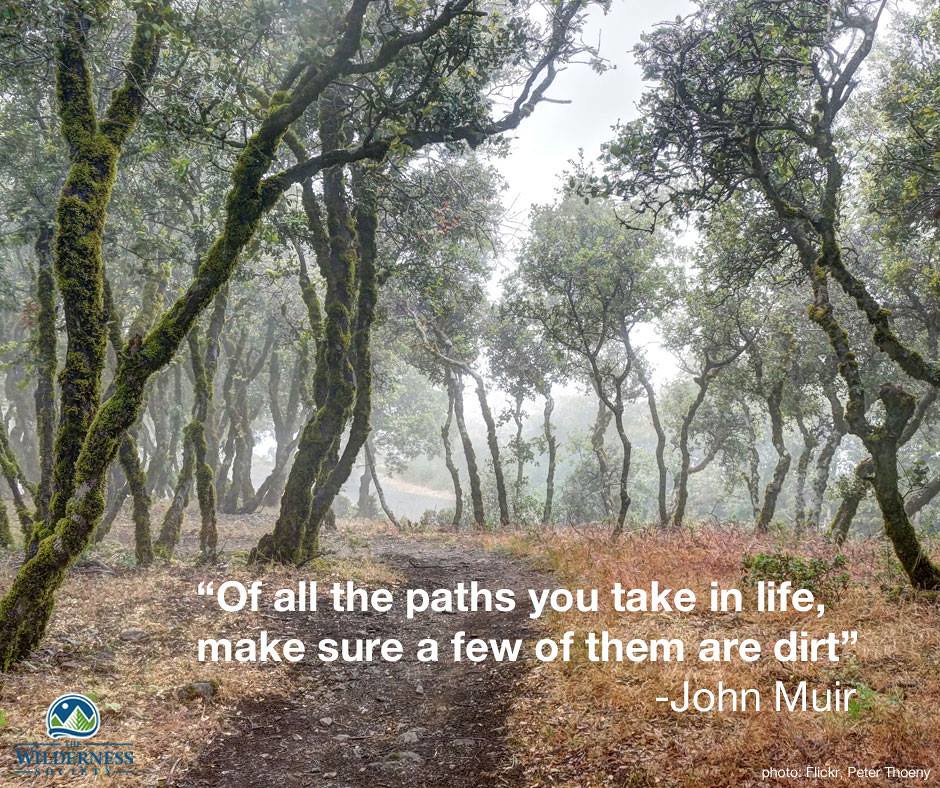The photo captures a serene, outdoor woodland scene, likely during late fall or early winter, characterized by a narrow, dirt path meandering through a forest of sparse, knurled tree trunks covered in moss. The trees, which are losing their leaves, giving the impression of an open, airy wood with most of the foliage concentrated at the top, create a slightly gloomy ambiance. The forest floor is strewn with dried brownish-orange grass, leaves, and scrub brush, and the weather appears overcast, possibly foreshadowing rain or snow. An inspirational quote by John Muir adorns the bottom right of the image, stating, "Of all the paths you take in life, make sure a few of them are dirt." This quote is in white font. The bottom left features a circular logo with mountains and the word "Wilderness." Additionally, the bottom very right credits the photo to Peter Thione on Flickr.